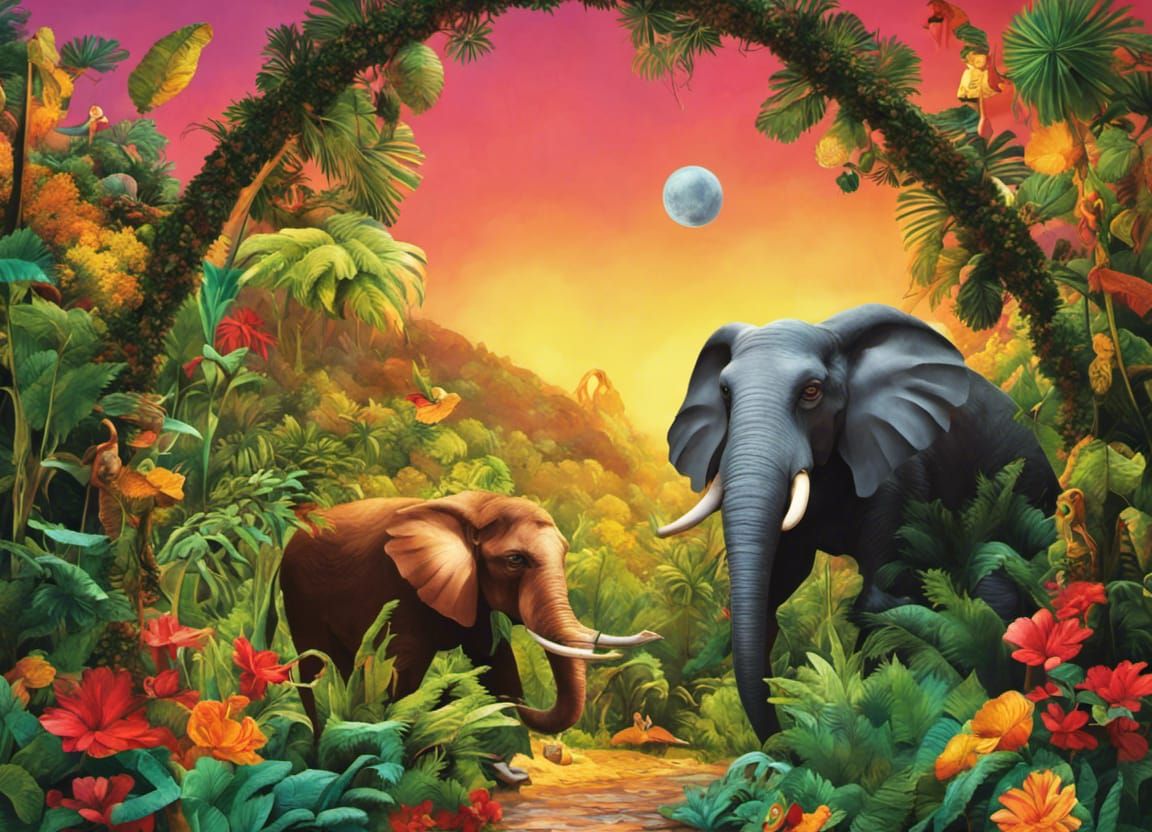The digital painting portrays two elephants standing in a jungle, surrounded by lush tropical plants and vibrant flowers. The larger elephant, a striking gray with white tusks, stands prominently beside a smaller brown elephant, also adorned with white tusks. These elephants exhibit a sense of melancholy, with their sad-eyed, expressionless faces. The scene is bathed in dominant hues of green and orange, with pink and orange flowers dotting the lush greenery at the bottom.

Above the elephants arches a verdant green wreath, framing the top of the image and drawing the eye towards a somber gray moon that hangs in a light peachy sky. The sky transitions from a soft pink at the top to a lighter yellow towards the bottom, creating an ethereal backdrop. This captivating jungle scene, though described by all as having an AI-generated feel, masterfully blends surreal elements with a poignant and almost eerie atmosphere.